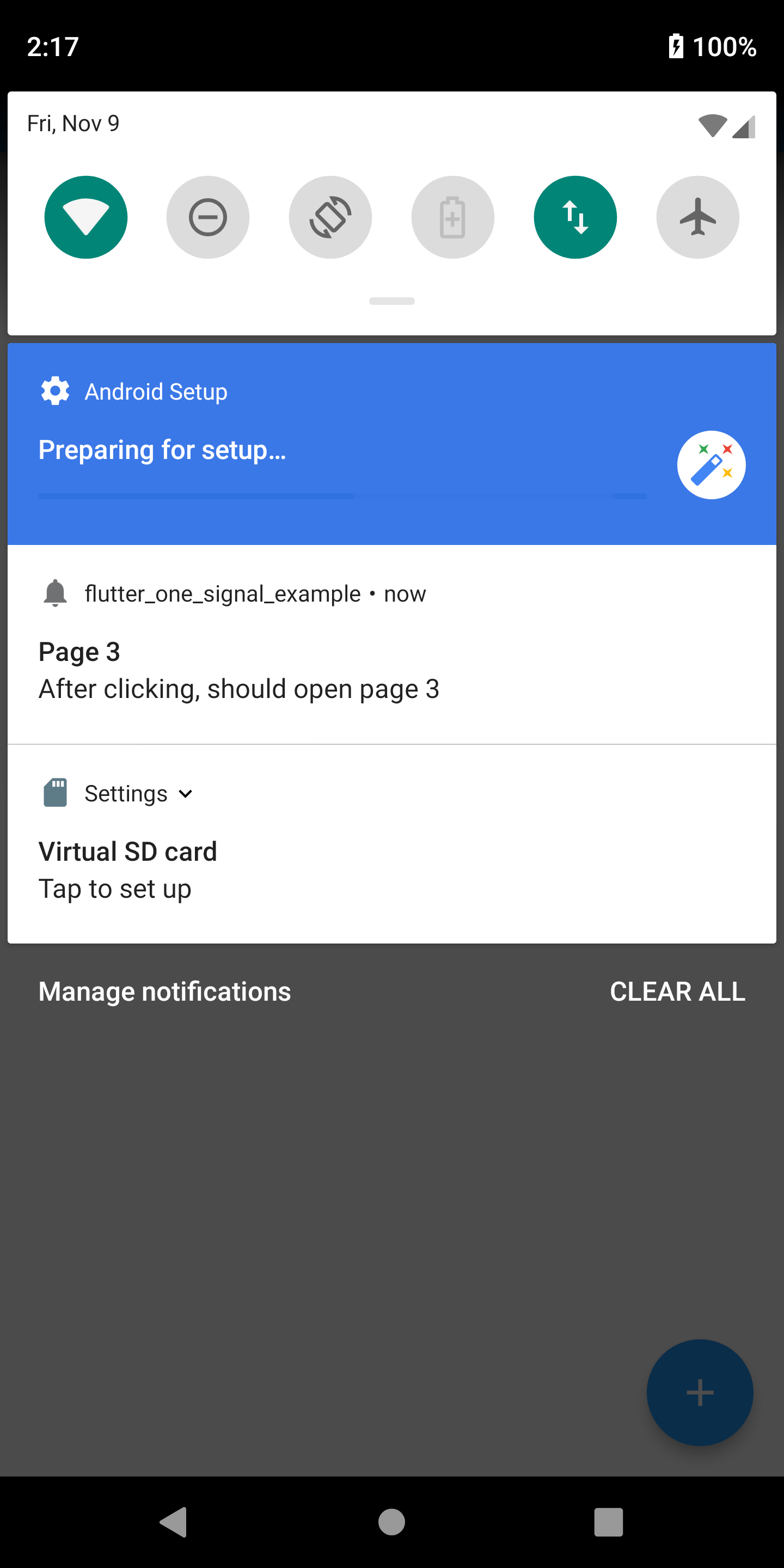The image displays a smartphone's notification center that has been pulled down. At the top of the screen, the time is displayed on the left as 2:17, while on the right, a battery icon shows it is fully charged at 100% and currently charging. The icons at the top are white against a black background.

Directly below, the notification center itself has a white background and displays the date as Friday, November 9. Several quick access icons are visible: Wi-Fi is selected and highlighted in green and white. The "Do Not Disturb," "Auto Rotate/Lock Rotation," "Battery Saver," and "Airplane" icons are present but not selected. Mobile data is selected and also highlighted in green and white.

Moving further down, there is a blue notification text stating "Android setup" with a message "Preparing for setup," accompanied by a gear icon for settings. Below this, another notification with a white background reads "Flutter 1 signal example" with the text "Now page 3. After clicking should open page 3." The final notification displays a picture of an SD card and the text "Settings" followed by "Virtual SD card. Tap to set up."

At the bottom of the notification panel, there is an option to "Manage notifications" in white text. Towards the bottom right, "Clear all" is written, which likely serves as a button to remove all notifications. The very bottom part of the screen features a dark background with a blue plus button located at the bottom right corner.